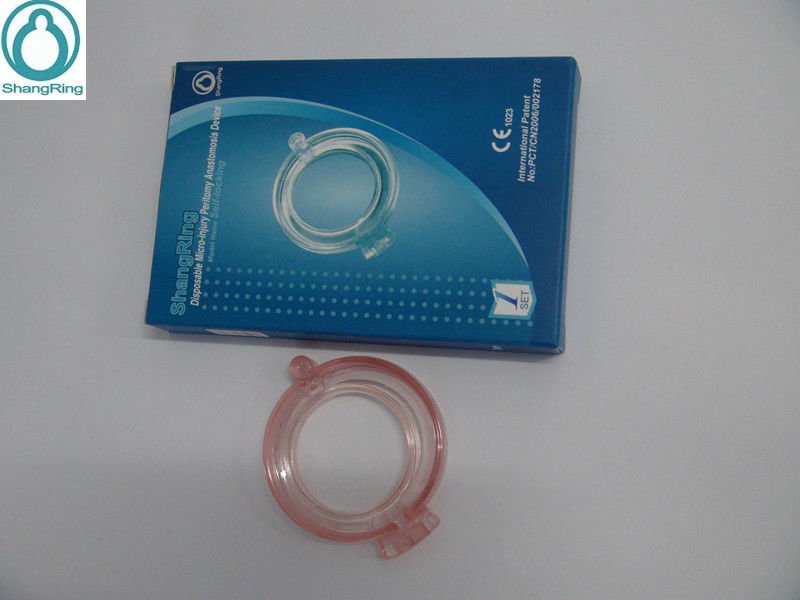The image depicts a blue rectangular box and its contents, contrasting the packaging and the item itself. At the top left corner of the box, in teal-colored letters, it reads "Shang Ring" alongside a symbol. The box is labeled "Shang Ring Disposable Micro-Injury Peritoneal Anastomosis Device" and indicates "one set." The exterior of the box features a design with arcs in different blue shades. The device, visible outside of the box, is a pink-tinged, translucent circular plastic ring. It is not a simple round ring but includes a rectangular attachment on one side and a rounded nodule opposite it.